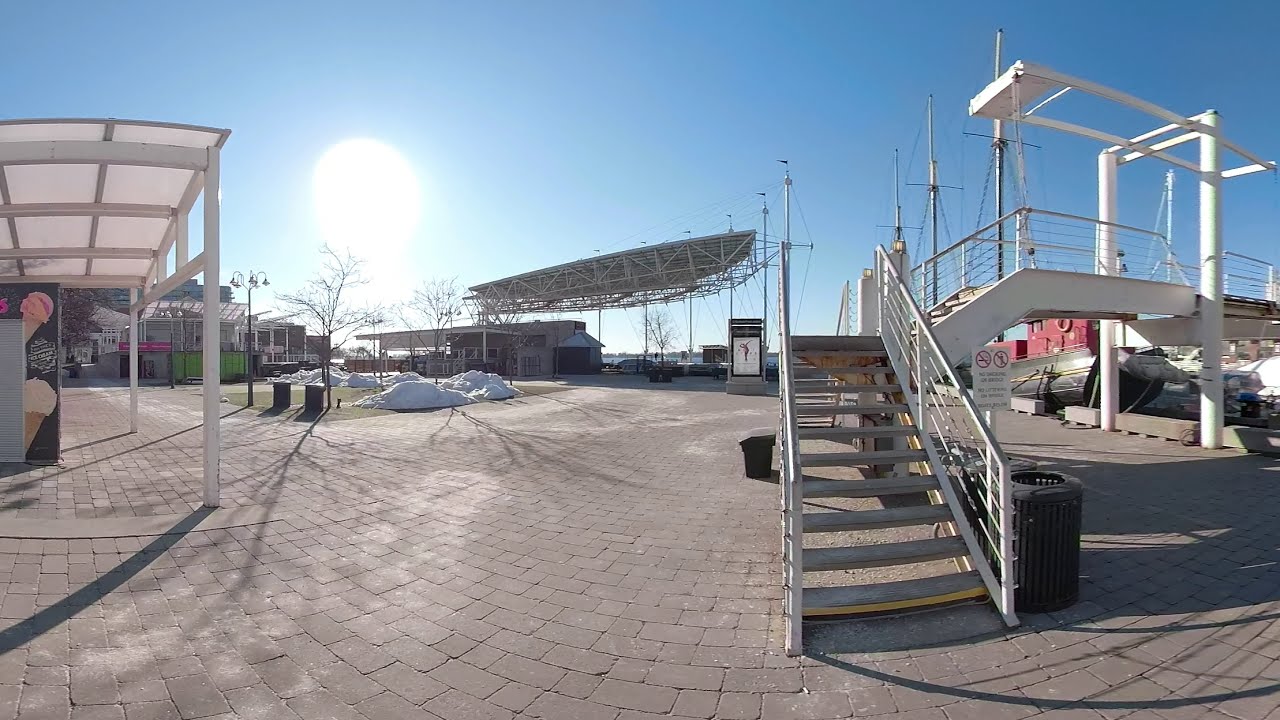A panoramic photograph captures a dock area under a brilliant, cloudless blue sky with the blazing white sun visible on the left. Dominating the right side of the image are a set of stairs, leading to more stairs and possibly a bridge, with small boats, including a notable red and black tugboat, positioned behind. The center of the frame is occupied by a white building, adorned with a mural and flanked by mounds of snow, with some elements suggesting stadium structures in the distance. To the left, a row of shops and buildings with a canopy overhead is visible. An ice cream vending machine is prominently featured on this side. The ground below consists of dark gray concrete bricks. Overall, the area appears somewhat empty yet tailored for tourists, evoking a blend of beach and park vibes, with a small grassy patch, some trash cans, trees, and signage typically found in a lifeguard-monitored zone.